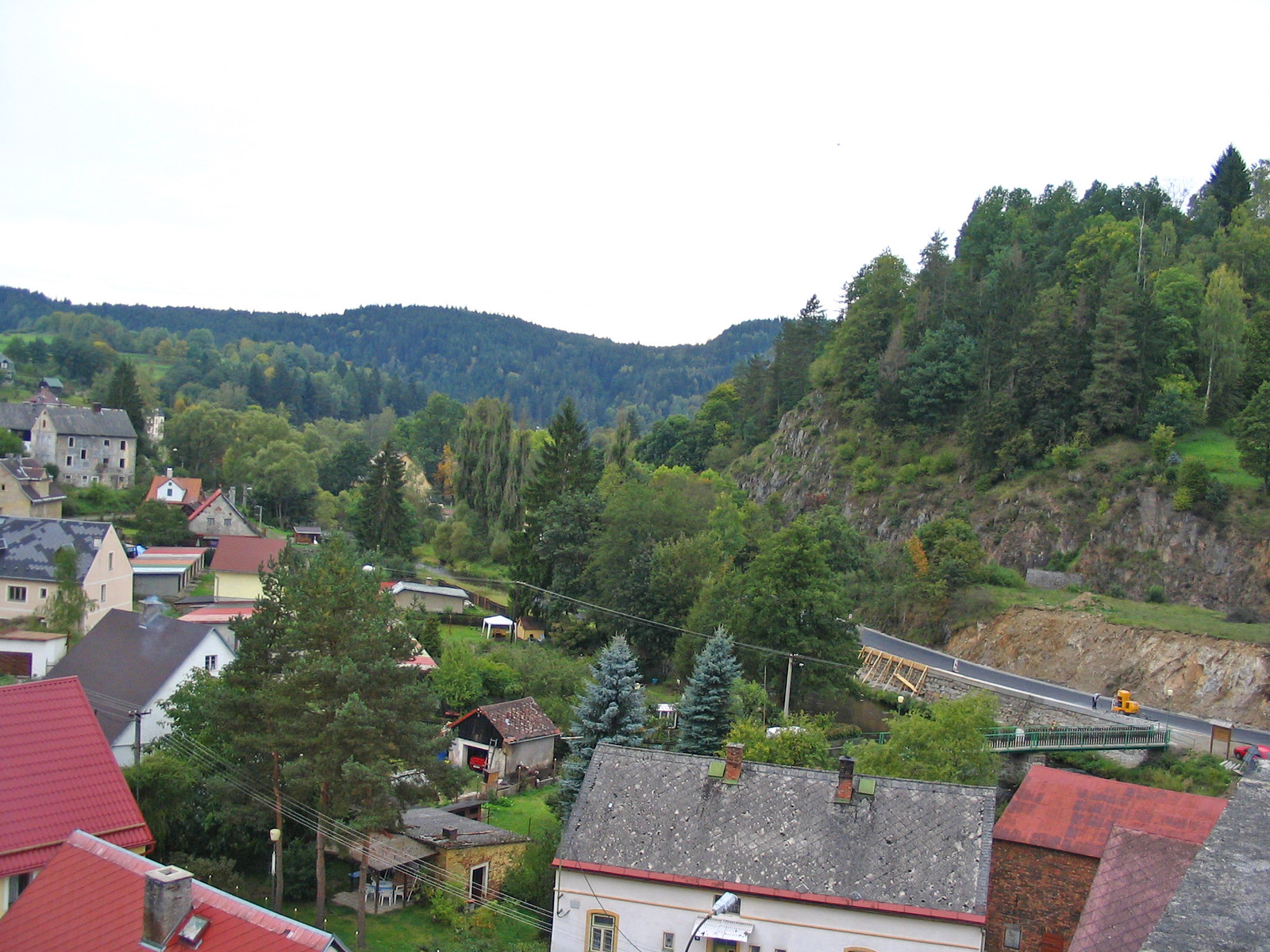The photograph depicts a serene hillside village viewed from an elevated perspective, capturing both the natural and residential elements of the area. Dominating the right side of the image is a hill with a rocky face, crowned with pine trees. Below this, a road winds its way through the landscape, marked by a yellow traffic light and various signs, hinting at a red car traveling along its path. The left side of the image is filled with a cluster of small stucco houses, their roofs varying from shades of red and orange to dark brown and grey. The roofs intersperse with patches of greenery, revealing sheds and power lines among them. The distant background reveals more low hills and trees, shrouded in a hazy, overcast ambiance, adding to the sleepy, tranquil atmosphere of the village.